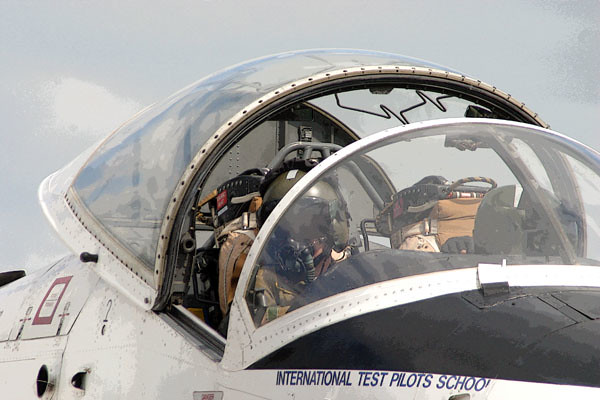The photograph depicts a close-up of the cockpit of an aircraft associated with the International Test Pilots School, identified by blue lettering partially visible on the lower part of the jet. This black and white aircraft has its nose cut off from the frame. A male pilot is seated inside, wearing an olive green helmet connected to a breathing apparatus, necessary for maintaining respiration once the cockpit canopy, currently partially open by about two feet, is fully closed. He is looking towards the right side of the plane, where the camera is positioned, and is gripping a lever or button. The cockpit lacks a co-pilot, and a backpack is visible in the seat. An unreadable red square sign and other minor details are visible on the jet's side panel. The scene captures an overcast, grey day, with portions of the light blue sky and cloud cover visible in the background.